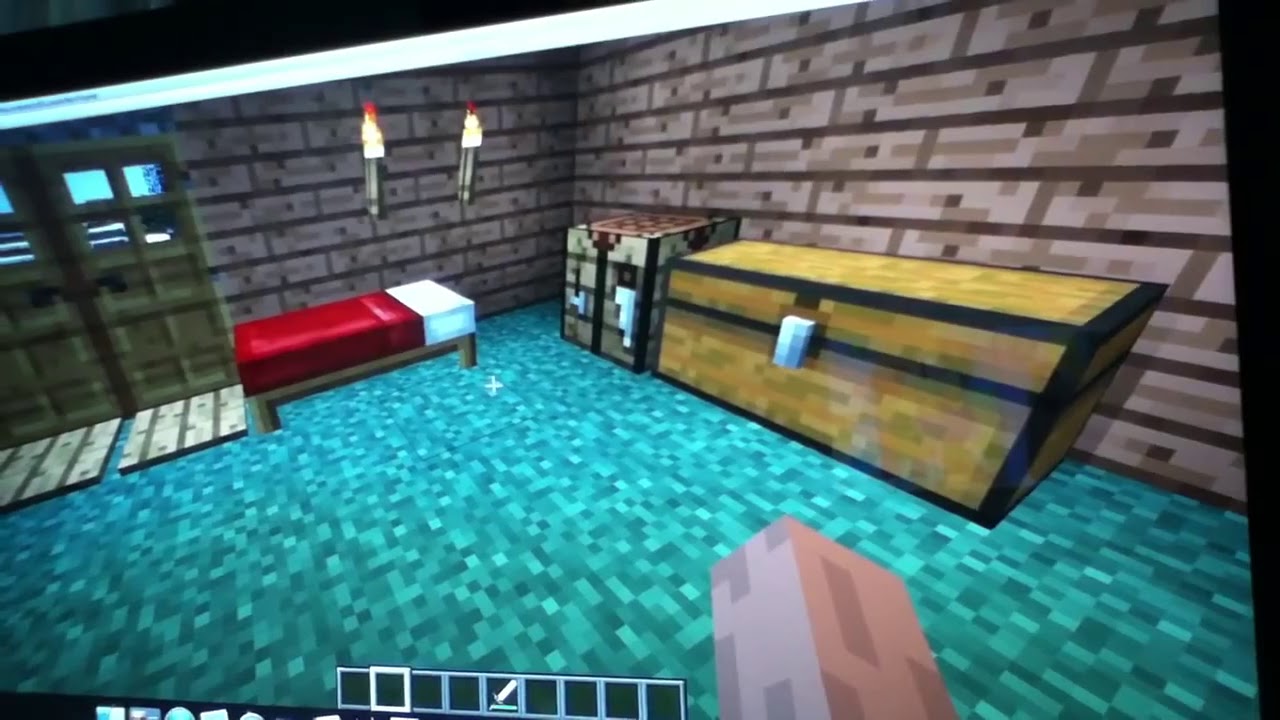The image is a screen grab from the video game Minecraft, showcasing the in-game inventory UI at the bottom of the screen. The inventory is mostly empty with four vacant squares, a sword icon with a green bar indicating its durability, and four additional green squares in a row. The player appears to be inside a self-constructed wooden building. The floor is a light green hue, and the room contains several key furnishings: in front of the character, there is a long brown chest with black edging, a square crafting table, and to the left of the crafting table is a bed with a brown frame, red sheets, and a white pillow. Above the bed, two lit fire torches are mounted on the wall. The walls of the room are composed of gray stones arranged in a brick pattern. Additionally, large green doors with four small windows at the top and black handles are visible to the left and at the back of the image, suggesting a castle-like environment. The overall aesthetic is characterized by Minecraft's signature block style.